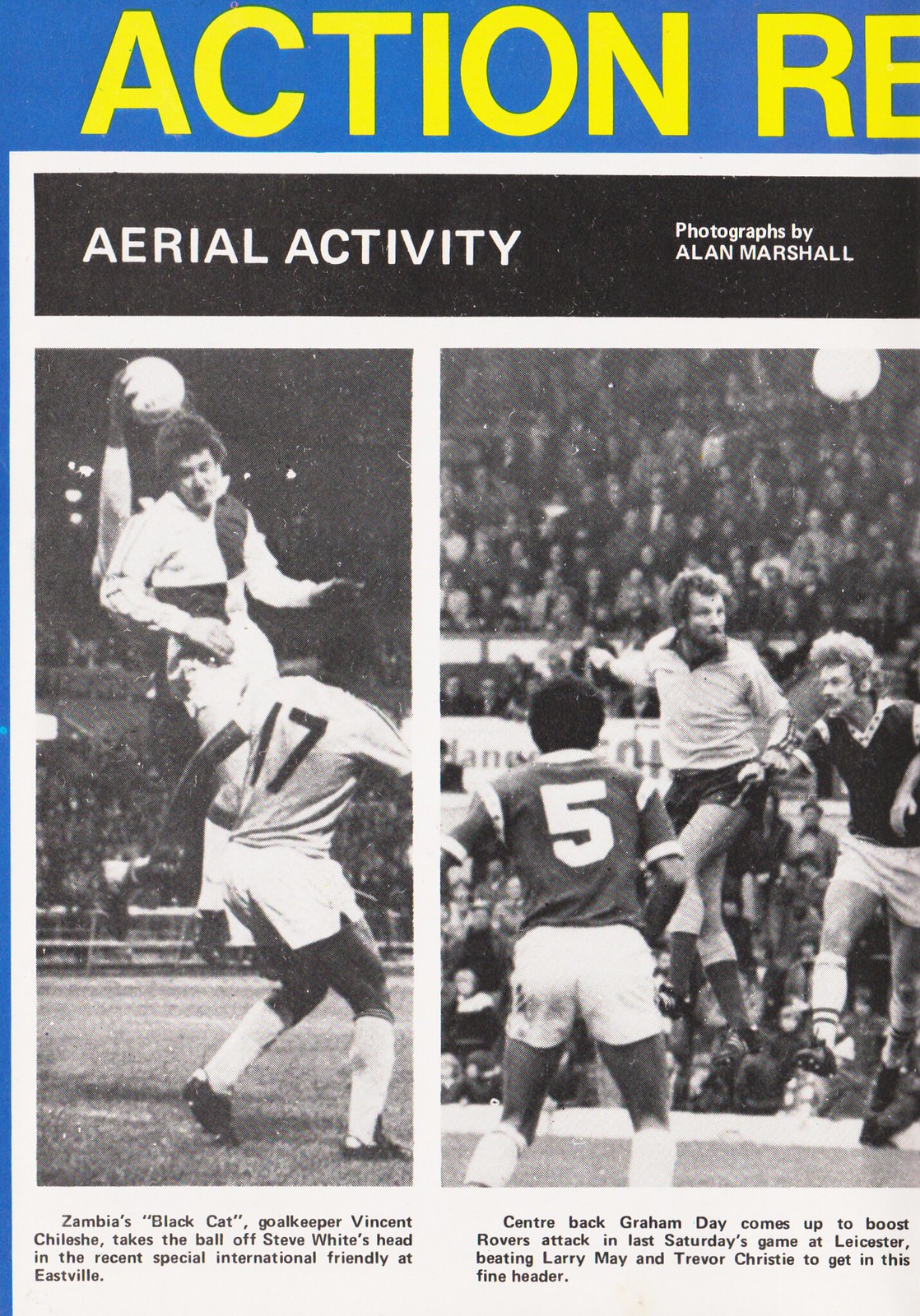This vertical-rectangular image, resembling a section of a vintage newspaper or soccer club program, features a portrait orientation with a predominantly black-and-white design accented by spot color. At the very top, a partially visible dark blue horizontal band spans the image, featuring bold yellow letters that read "ACTION RE", though the full text is cut off. Below, a complete black band stretches across with the white text "AERIAL ACTIVITY", and a photographer credit is present.

Situated beneath are two black-and-white photographs capturing dynamic moments from a soccer game, each accompanied by descriptive captions. The photograph on the left depicts Zambia's black-capped goalkeeper, Vincent Jules Gillespie, skillfully intercepting the ball from Steven White's head during a recent Special International Friendly at Eastville. The action shot prominently displays the players mid-air with the soccer ball visible. The right photograph features center back William Day soaring between two opposing players, Larry May and Trevor Christie, in a dramatic aerial duel. Day, wearing a white jersey and dark shorts, beats the opposing team players, clad in dark jerseys and white shorts, to the ball, which is positioned in the top right corner of the image. The caption highlights his effort to propel Robles' attack in the final moments of the game against Lester. This composition is framed on the left by a vertical blue rule, enhancing the vintage feel of the entire layout.